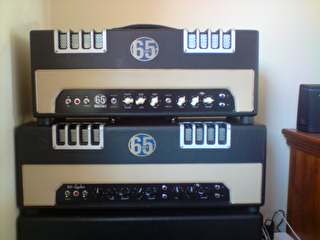The photo showcases an indoor scene featuring a white wall and a wooden dresser or shelf on the right side of the frame, bearing a black object. Central to the image are two identical, rectangular electronic devices stacked on top of each other, resembling the back end of sophisticated audio-visual equipment such as DVD or Blu-ray players. Each device is characterized by a split color scheme—with the top half in gray and the bottom in cream— and prominently displays the number 65 in a silver circle on a darker gray background. Flanking this number, there are metal grates or vents on the upper left and right, possibly for cooling. A series of dials, knobs, and various colored input jacks are visible at the bottom, suggesting multiple connectivity options. The two devices rest on a black shelf, and a few cords can be seen trailing between them. Overall, the setup looks functional and geared toward high-end electronic usage.